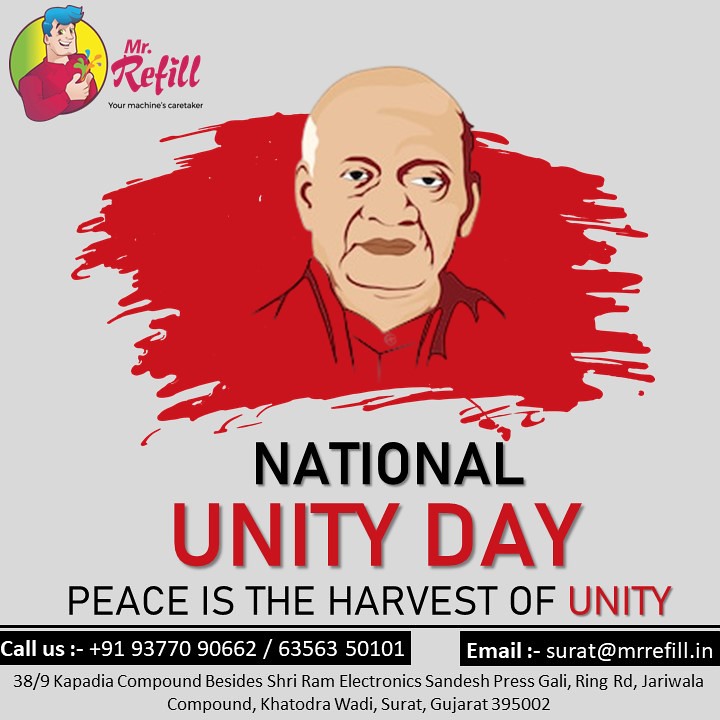This digitally generated advertisement poster features a light gray background with a striking red brushstroke swath in the center, showcasing a detailed ink drawing of an elderly bald man with white hair on one side. He is framed within the red paint, drawn in brown lines. The top left corner of the poster sports a colorful logo: a cartoon figure with blue hair, a red shirt, and a smile, set against a yellow circle, alongside the text "Mr. Refill" and the tagline "your machine's caretaker."

Below the central image of the elderly man, identified as Mr. Sardar Vallabhbhai Patel, an Indian leader, the headline "National Unity Day" stands out, with "National" in bold black letters and "Unity Day" in bold red letters. The subheading "Peace is the harvest of unity" is in black, with "unity" emphasized in red.

Toward the bottom, a black strip on the left provides contact numbers: +91 93770 90662 and 63563 50101. Opposite, another black strip lists the email address: surat@mrrefill.in. The footer includes an address in detailed text: "38/9 Kapadia Compound, besides Sriram Electronics, Sandesh Press Gali, Ring Road, Jariwala Compound, Kathodra Wadi, Surat, Gujarat 395002."